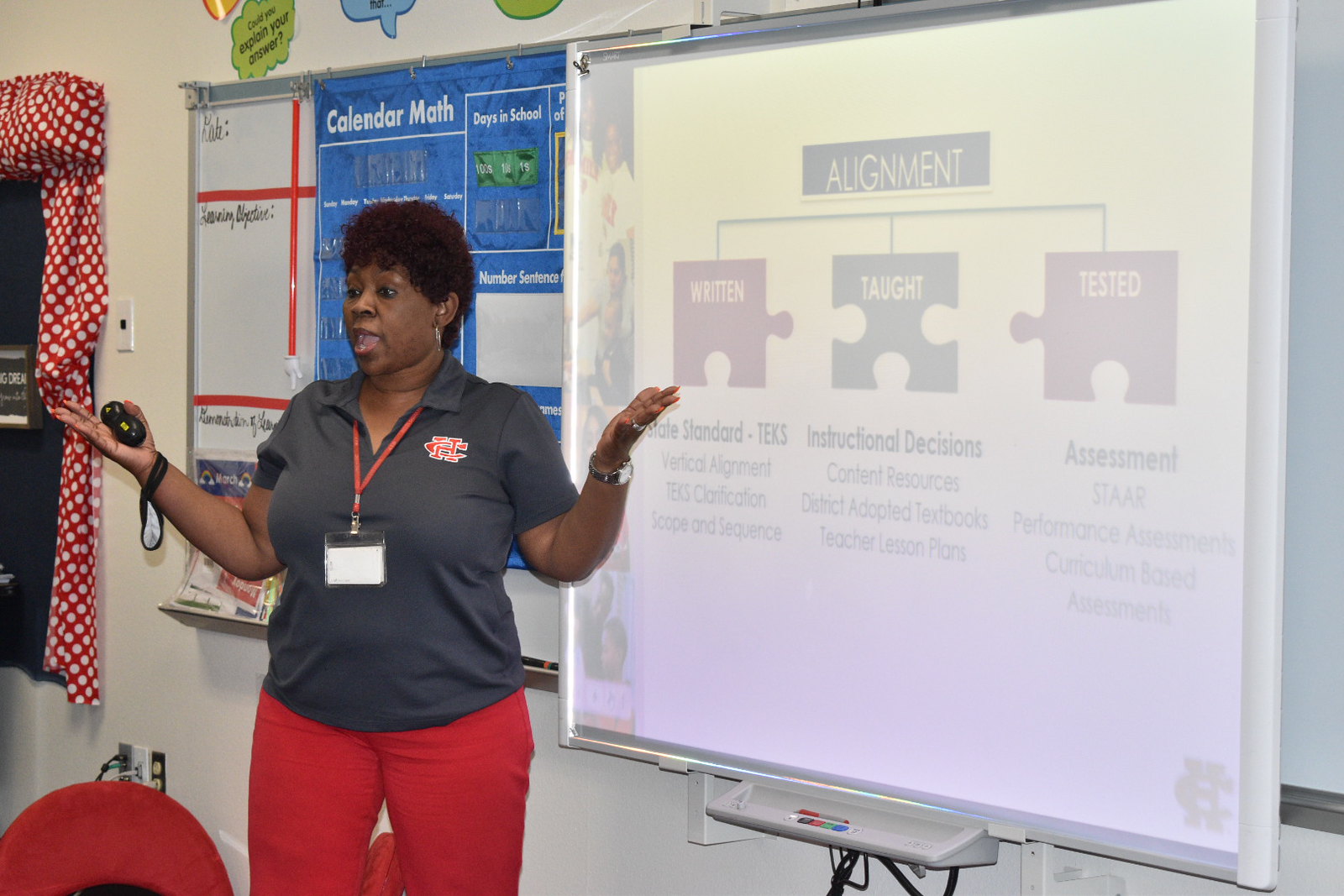The photograph depicts a black woman with short black hair, identifiable as a teacher, standing in a classroom. She appears engaged and in mid-instruction, holding a handheld remote with a strap in her right hand, and her arms spread out in an expressive manner. She is dressed in a logo-bearing gray polo shirt, red pants, a watch, rings, and a red lanyard with a white badge. Behind her, a large whiteboard displays a PowerPoint slide with the title "Alignment" and three interconnected puzzle pieces labeled "Written," "Taught," and "Tested." Each puzzle piece details specific educational elements such as "State Standard," "Instructional Decisions," and "Assessment." Other classroom materials include a "Calendar Math" sign, books, and markers. The setting features white walls, a red chair, an electrical outlet, a window adorned with red and white polka dot curtains, and a whiteboard with numerous instructional notes. The teacher's expressive posture and the detailed materials around her suggest she is deeply engaged in delivering an educational presentation to her unseen students.